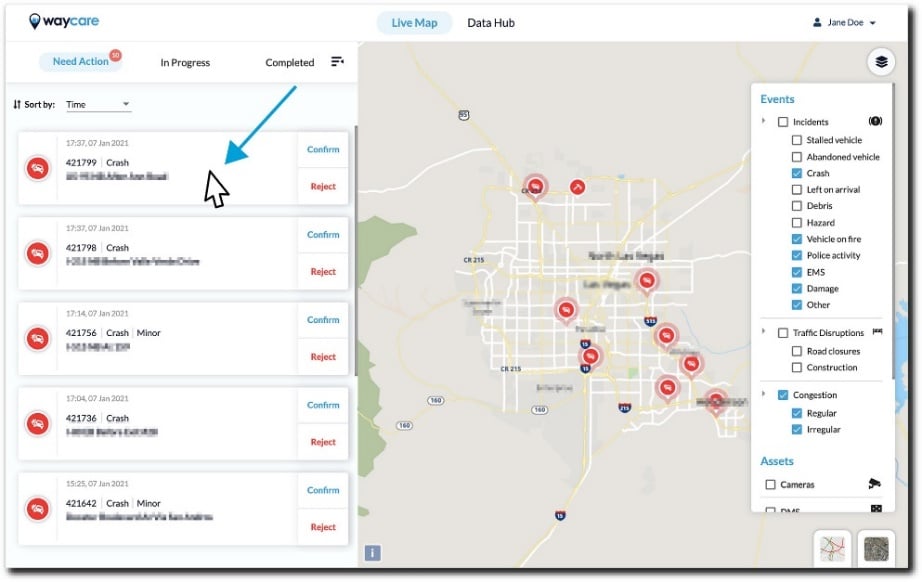In the top left corner of the image, there is a pin icon typical of map markers, featuring a black outline and a blue fill. Adjacent to it, the text "Waycare" is displayed, with "WAY" in black and "CARE" in light blue. Below this, a light gray-bordered area contains three options: "Need Action," "In Progress," and "Completed." "Need Action" is presented in blue font and is accompanied by a small orange circle with unreadable white text.

A downward-pointing arrow extends from "Completed" towards a listing. This listing includes a red circular icon with a white border and a car symbol in the center. At the top of the listing, "17:37, 07 JAN 2021" is written in gray text, followed by the bolder black text "421799." Below a light gray divider, the word "Crash" is displayed. There is another row of black text, but it is blurred out. To the right, two separate buttons labeled "Confirm" (in blue) and "Reject" (in red) are visible.

On the right side of the image, a map with a beige background showcases several roads marked in white, adorned with various pins, each with a red circle and car icon. Additionally, a white rectangular pop-up menu labeled "Events" is located at the top left of the map.